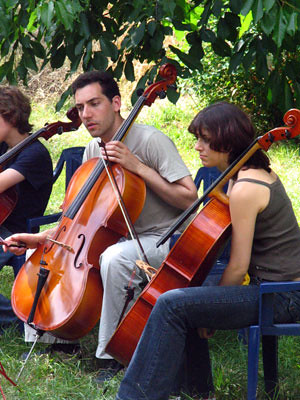In the photograph, three people are seated on blue plastic chairs in a park setting, surrounded by lush greenery. They are positioned under a tree with an abundance of leaves, some of which nearly brush the head of the man in the middle. All three individuals are holding cellos, resting their instruments on the grass-covered ground.

The woman on the right has dark brown hair cascading down her neck and wears a gray spaghetti strap top paired with blue jeans that flare at the bottom. She holds her cello in front of her, with a focused gaze likely directed at a music stand just out of view.

Next to her, the man in the center sports a tan, short-sleeved shirt and white tan pants. He also holds a cello, with the bow in his right hand and positioned slightly out of frame. His dark brown hair contrasts with the green foliage behind him.

On the far left sits another individual, dressed in a dark blue-purple short-sleeved shirt and blue jeans. Like the others, he has a cello propped in front of him as he sits under the tree’s leafy canopy. Their coordinated posture and shared focus suggest they are engrossed in their musical performance amidst the serene park ambiance.